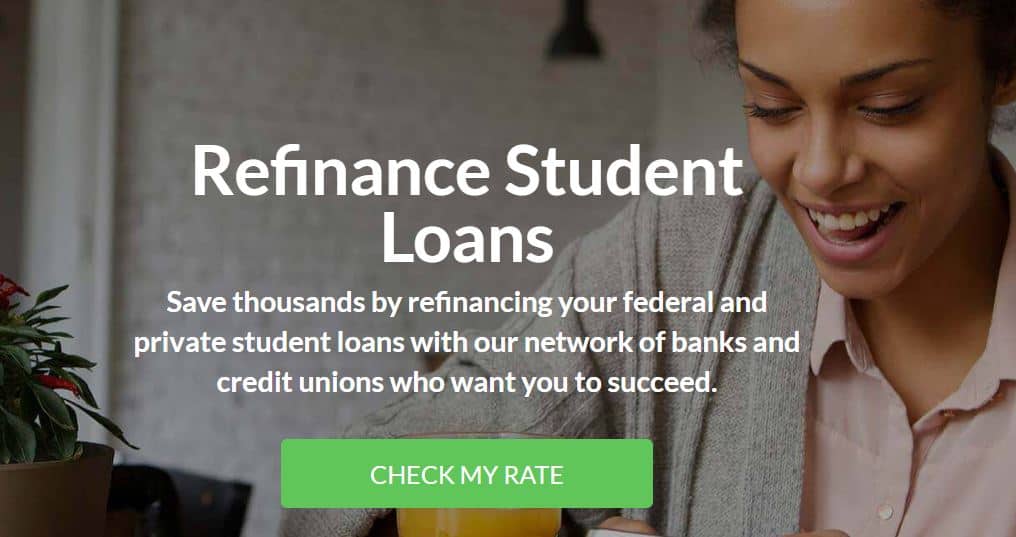This advertisement for refinancing student loans features an African-American woman on the right-hand side of the screen, dressed in a gray sweater layered over a pink shirt. The background is styled with a modern, black hanging pendant lamp, a coleus plant, and curtains against a neutral wall. Dominating the left side is bold white text that reads "Refinance Student Loans." Below that, in smaller text, it details the potential savings: "Save thousands by refinancing your federal and private student loans with our network of banks and credit unions who want you to succeed." A prominent green button at the bottom, with white uppercase letters, instructs viewers to "CHECK MY RATE." This call-to-action button directs users to another interface where they can input personal details to explore options for reducing their repayment burden by potentially lowering interest rates and refinancing both federal and private student loans through various financial institutions.